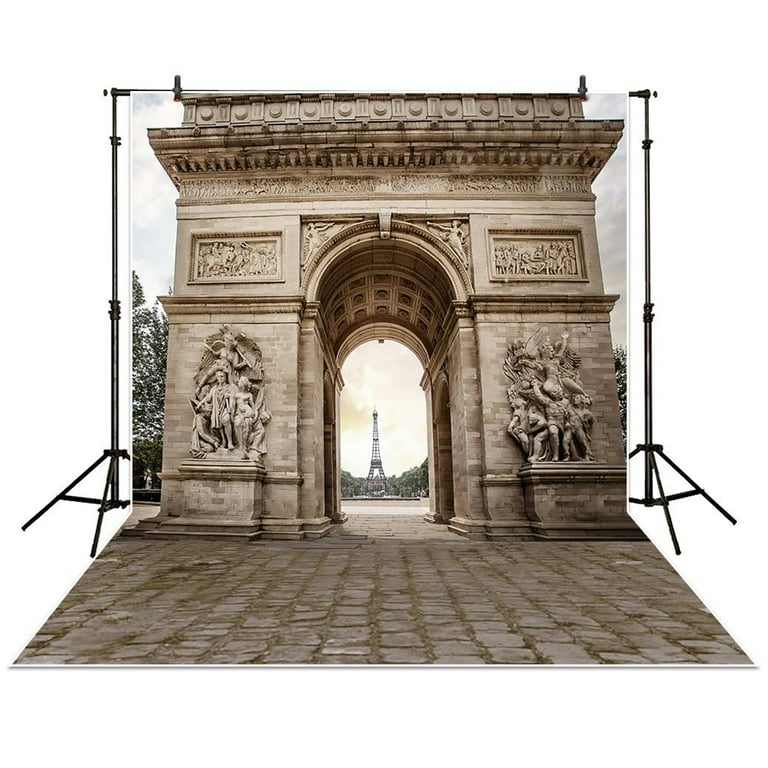The image depicts a detailed photographer's backdrop designed to replicate the Arc de Triomphe in Paris. This large cloth backdrop, hung from a black bar supported by two tripod-like stands, extends all the way to the floor, creating a seamless scene for photography. The backdrop features meticulous details, including the iconic archway, sculpted reliefs of angels and people, and the platform above the arch. The intricate sculpted areas under the archway can also be observed. Through the archway, the Eiffel Tower is visible in the distance, surrounded by clouds and green trees at its base, suggesting an outdoor setting. The backdrop rests on a cobblestone-like ground that extends to the floor, enhancing the realism of the scene. The sides of the image reveal a cloudy blue sky, reinforcing the illusion of an open, outdoor environment.